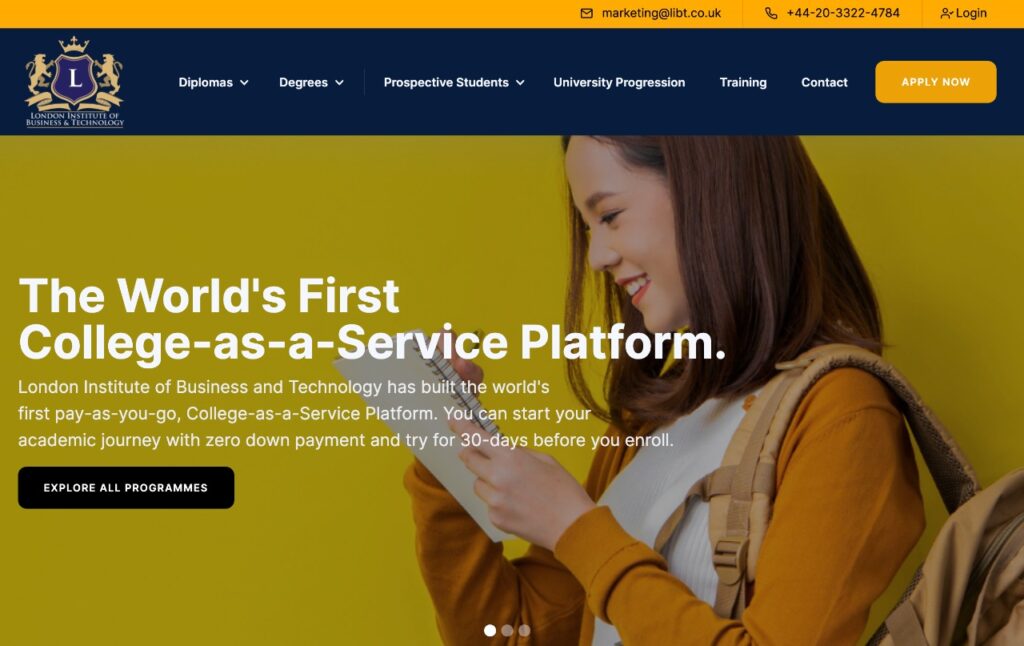At the top of the image, there is a prominent yellow banner with black text on the right-hand side. Within the banner, there's an icon of a mail envelope followed by the email address "marketing@ibt.co.uk". Additionally, a phone icon is displayed alongside the number "+44 203 322 4784". Also present is an icon of a person next to the word "Login".

Beneath the yellow banner, the next section features a black background. On the left side, there is a distinguished logo consisting of two gold lines with a crown on top, and a blue crest emblazoned with a white letter 'L'. Beside the logo, the text reads "London Institute of Business and Technology." 

This section is followed by a series of clickable links that include options such as "Diplomas," "Degrees," "Prospective Students," "University Progression," "Training," and "Contact." There is also a yellow square with white text that reads "Apply Now."

On the right side of this section, set against a green background, there is an image of a woman of Asian descent with dark brown hair. She is gazing to the left at a notebook she holds in her hand. She is dressed in a white shirt paired with a green long-sleeve open shirt and has a tan backpack slung over her shoulder. 

In the bottom right corner of this section, white text proclaims, "The world's first college-as-a-service program. London Institute of Business and Technology has built the world's first pay-as-you-go college-as-a-service program. You can start your academic journey with zero down payment and try for 30 days before you enroll." Below this, there is a prominent blue button labeled "Explore All Programs," flanked by a white button in the center and two gray buttons on either side.